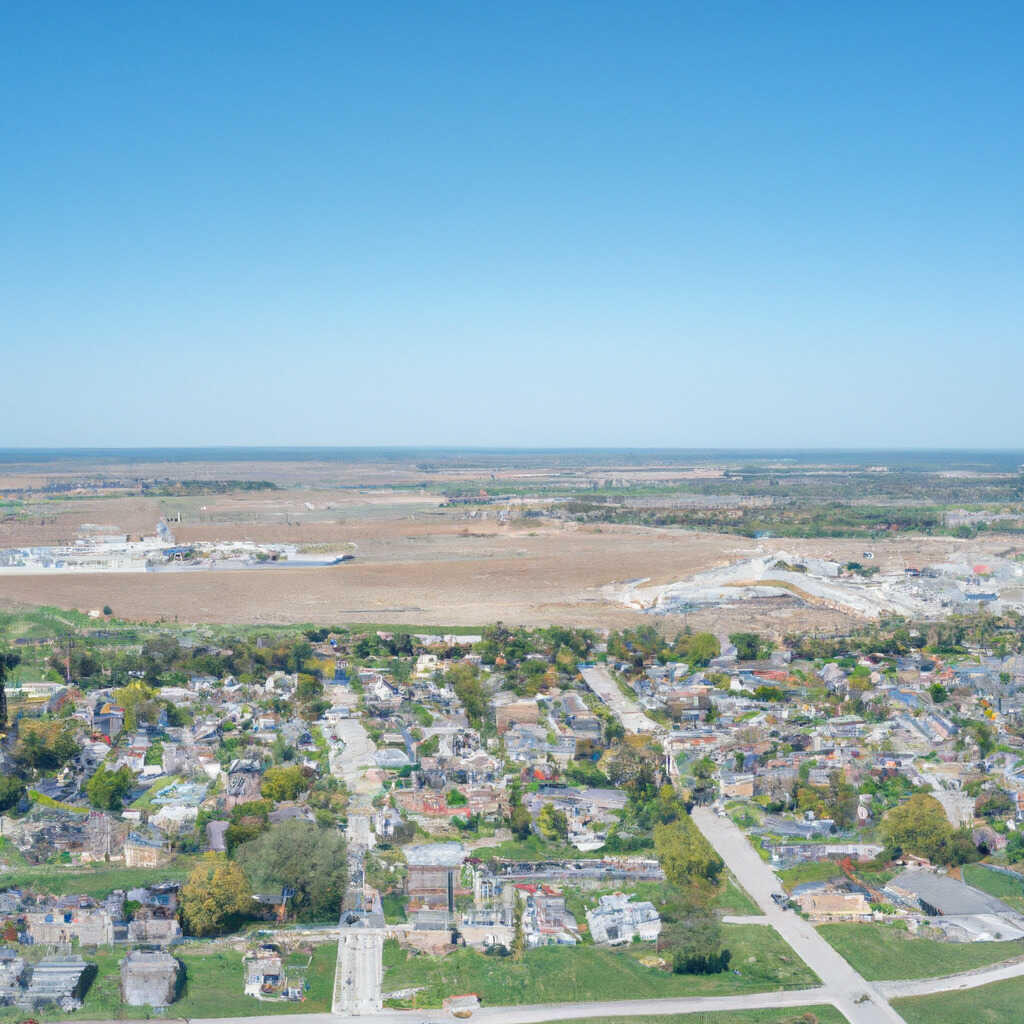This aerial view captures a small, flat landscape under a bright, cloudless blue sky. Dominating the foreground is a residential neighborhood with numerous houses, tree-lined streets, and patches of green grass in the yards throughout. The layout of this neighborhood seems to follow two main highways. Interspersed among the homes are commercial buildings, hinting at a small but possibly once vibrant community.

In the backdrop, the landscape transitions to more barren land, indicating a rural setting with fewer structures. To the right and further back, there are visible signs of industrial areas, including two large deteriorating factories showing significant rust and dilapidation, contributing to an abandoned look to parts of the city. Between these industrial zones lies a large expanse of open land, sparsely dotted with trees and bushes. The overall scenery suggests a place that, while bright and clear, holds a mix of thriving residential life and areas of industrial decay.